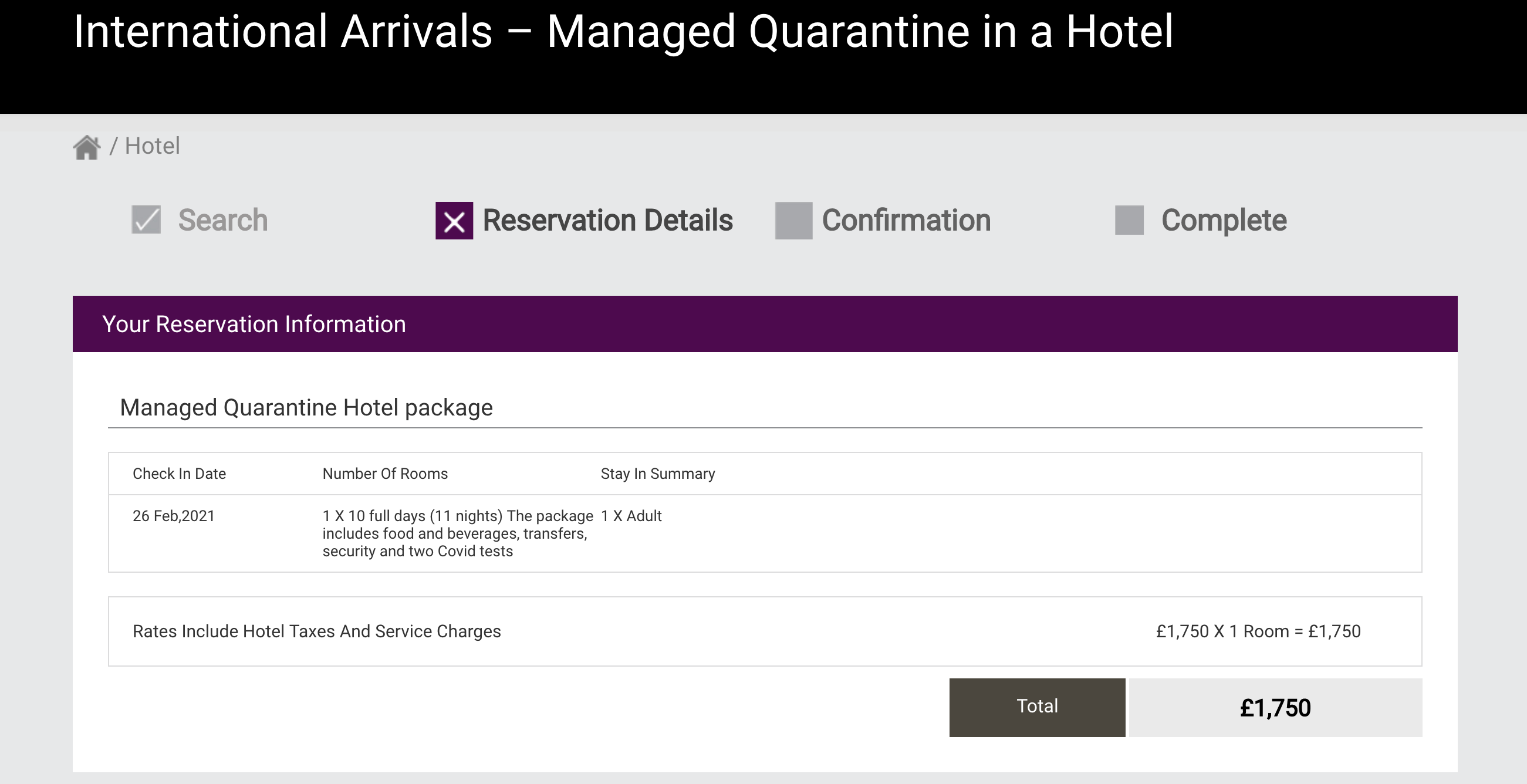Here is your cleaned-up and detailed caption:

---

The image displays a webpage on a computer screen detailing information about international arrivals and managed quarantine in a hotel. At the top, in white print on a black rectangle, the header reads "International Arrivals - Managed Quarantine in a Hotel." Below this, there is an icon of a house followed by a slash and the word "hotel."

Further down, a search check mark is shown followed by a purple box with an "X" labeled "Reservation Details." Next to this, a gray box labeled "Confirmation" is seen, followed by another gray box labeled "Complete." Beside each of these words, there are squares for check marks indicating stages of the process.

Beneath these navigation elements, a deep purple (almost black-purple) section contains text in white and purple. The white text reads "Your Reservation Information," followed by "Managed Quarantine Hotel Package." Detailed information below includes: 
- Check-in Date: February 26, 2021
- Number of Rooms: 1
- Duration: 10 full days, 11 nights

A further breakdown of the stay mentions "Stay Summary: 1 Adult," and specifies that rates include hotel taxes and service charges. The total cost for the package is highlighted as £1,750.

---

This refined caption maintains the detailed information provided and organizes it in a clear, structured manner.